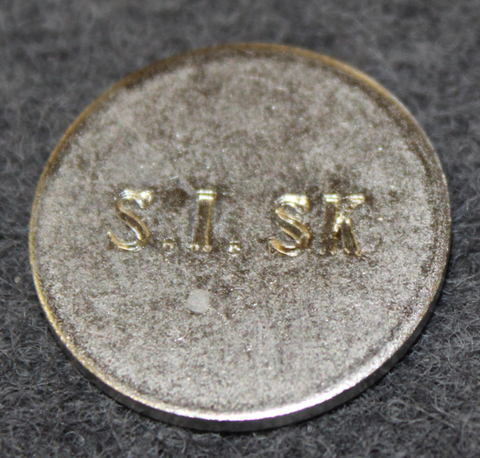The image depicts a single circular metallic object situated diagonally at the center of a fuzzy, gray fabric, likely wool or felt, which hints at a cozy domestic setting. The object—either a hobbyist or collector's coin, or possibly a branded button—stands out with its distinct metallic colors: a shiny, goldish hue along its smooth edges and a more rustic, rough center. The only text visible on the disc is the stamped letters "S.I.SK" in its shinier central area, indicating it may not be a real currency but rather a specialized or collectible item. The focus of the photograph captures both the intricate texture of the fabric and the contrasting metallic sheen of the disc.